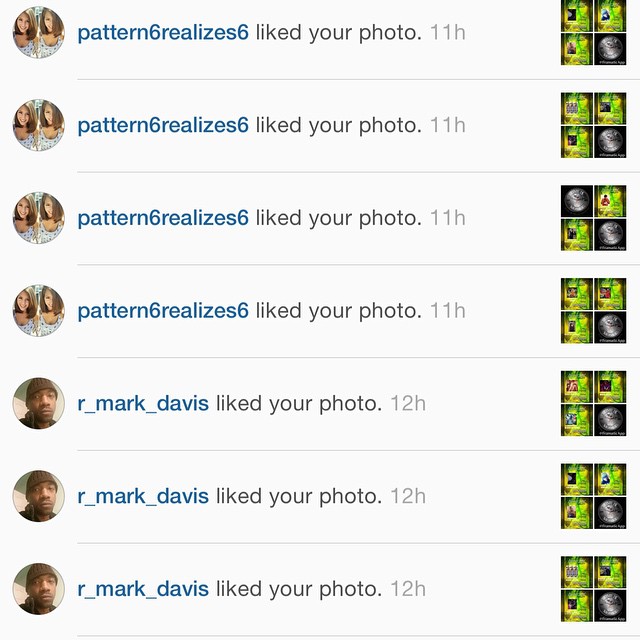The image displays a series of Facebook notifications showcasing recent likes on a user's photo. The notifications are arranged vertically, with the first four showing, "Pattern6realizes6 liked your photo 11 hours ago," and the subsequent three stating, "R_mark_Davis liked your photo 12 hours ago." Each notification includes the profile pictures of the users, with Pattern6realizes6 depicted as a girl with straight light brown hair, while R_mark_Davis is a young black man wearing a brown beanie. To the right of these notifications are a series of seven image grids, each consisting of four smaller pictures. These images vary, with some displaying green backgrounds and others a black background featuring a silver circle. The content appears to be some form of meme with distinct visuals in each quadrant of the grid.